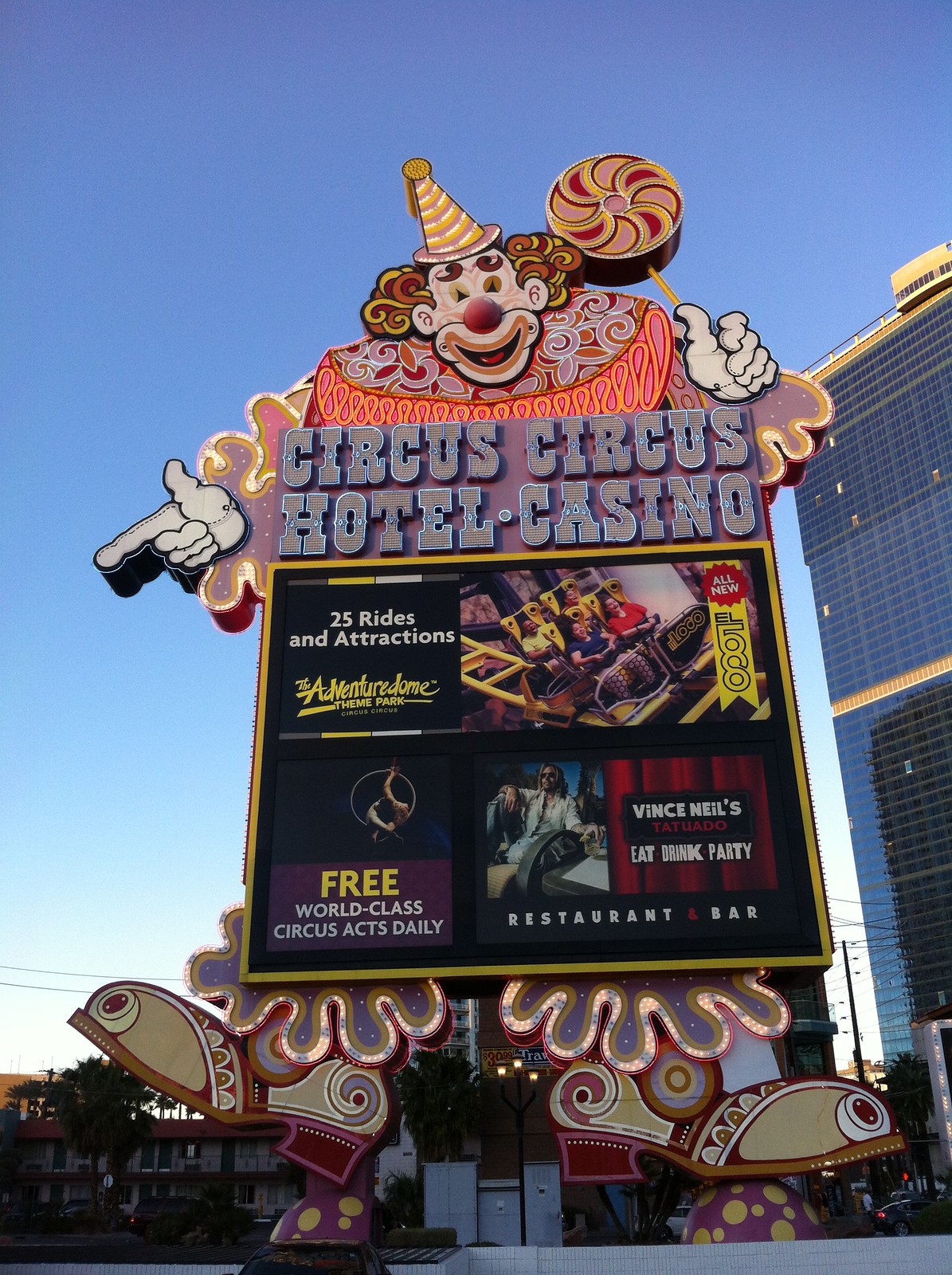In this daytime outdoor image, a large, elaborate sign stands prominently in the center, shaped like a clown, advertising the Circus Circus Hotel and Casino. The clown, adorned with a red and yellow curly wig, a white face with a big red nose, and a pink tongue visible in its half-open mouth, wears a cone-shaped party hat and an inner tube-like scarf with squiggly purple and orange lines. The clown's left hand holds a pinwheel, and its right hand points downward like a gun. Clad in white gloves and enormous clown shoes, the figure captivates attention. Text on the sign promotes the hotel's amenities, including "25 Rides and Attractions" and "Free World Class Circus Acts Daily," with mention of the Adventure Dome theme park and advertisements for Finn Sneil's Tattoo. The background reveals a clear blue sky, multiple buildings, including low-hanging structures at the bottom, a tall building with glass windows to the right, and surrounding vegetation with trees and grass. The scene vividly captures the bustling, whimsical essence of the casino's exterior.